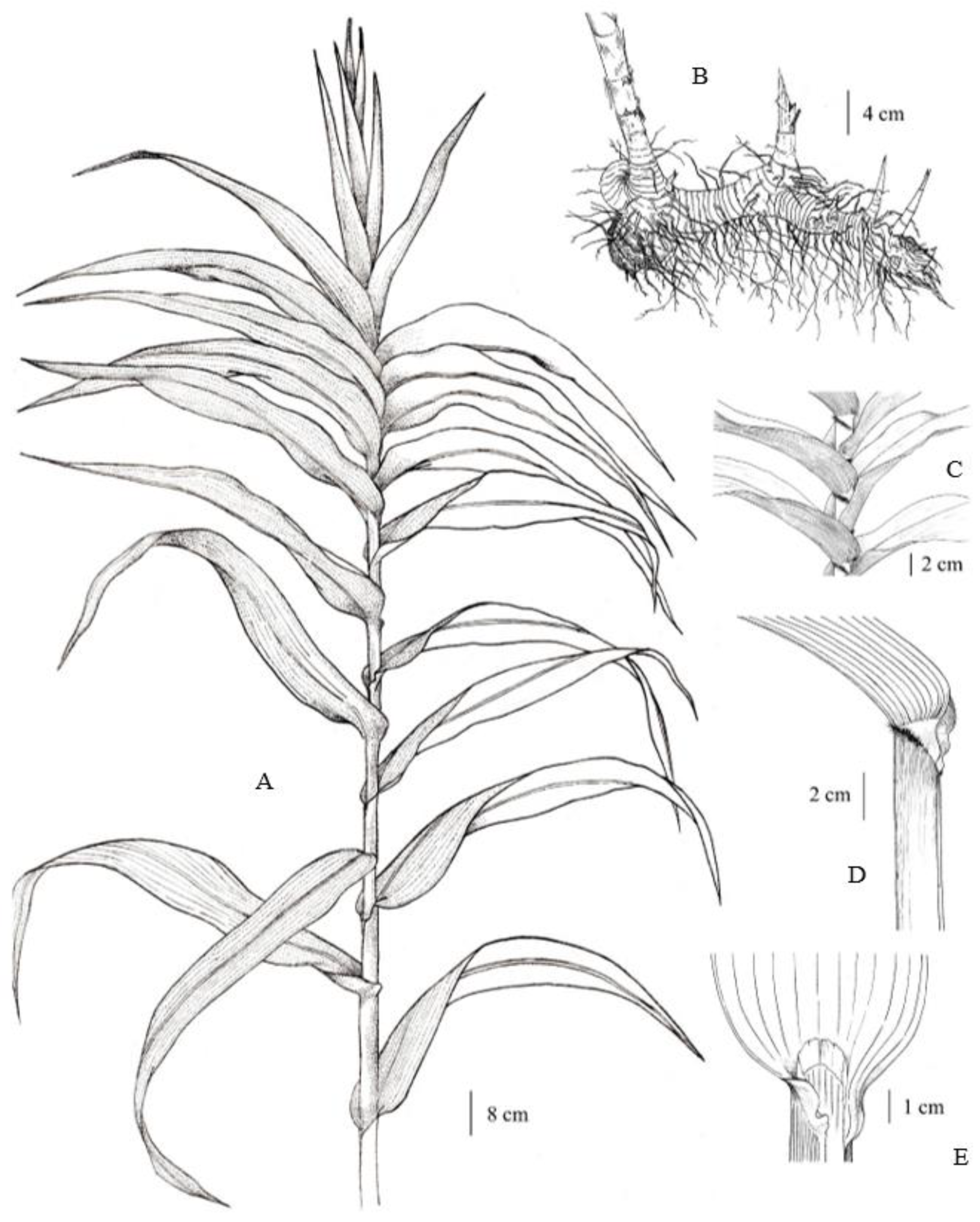This detailed botanical illustration features a vertically oriented pen and ink drawing of a tall plant with long, slender leaves arranged alternately along a central stem, increasing in density toward the top. The main image, labeled A, shows the full plant with a scale marking of 8 centimeters. To the right, a series of detailed close-ups break down parts of the plant:

- **Image B** reveals the fine, hairy root system branching from a thicker primary root, with a scale of 4 centimeters.
- **Image C** demonstrates the manner in which the leaves grow in an overlapping pattern along the stem, scaled to 2 centimeters.
- **Image D** focuses on a close-up of a leaf as it attaches to the stem, also labeled with a 2-centimeter scale.
- **Image E** provides an extremely detailed view of the leaf emerging from the stem, showing intricate textures and structure, scaled to 1 centimeter, located at the bottom right-hand corner.

The precision and arrangement of these labeled illustrations suggest it is likely from a scientific botany manual, meticulously detailing the structural characteristics and growth patterns of the plant.